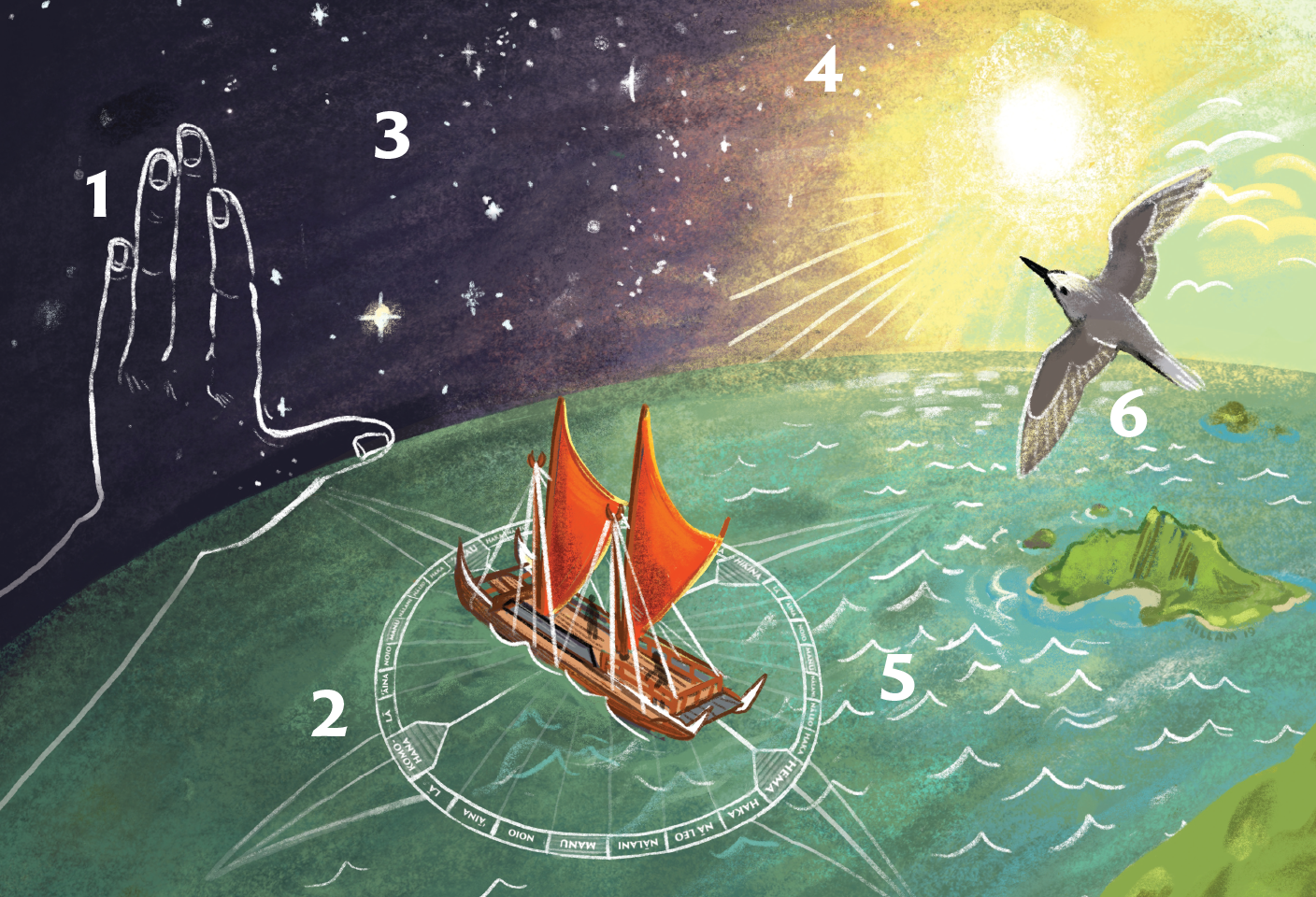The image is an animated and detailed painting serving both as a diagram and a method of navigation, potentially depicting how one might tell the day or time while on a boat. The illustration offers multiple steps or phases, with prominent numbers 1 through 6 marking different elements. In the upper left is a large numeral "1" adjacent to the silhouette of a left hand, fingers pointed skyward with the thumb extended outward, resembling an "L" shape. A red sailboat, marked with "2," navigates an ocean depicted within a circular frame, angled to show Earth’s curvature predominantly covered in water with minimal land. Number "3" is positioned in the sky to the right of "1," indicating astrological navigation by stars. The "4" is centered middle-right, next to the sun cresting over the horizon, indicating solar navigation cues. Number "5" hovers over the ocean in the middle-right, while number "6" is nearby, associated with a white swallow bird flying near a small green island. A comprehensive navigational diagram encircles the boat, detailing cardinal directions and aiding in holistic navigation using the sun, stars, and natural elements.